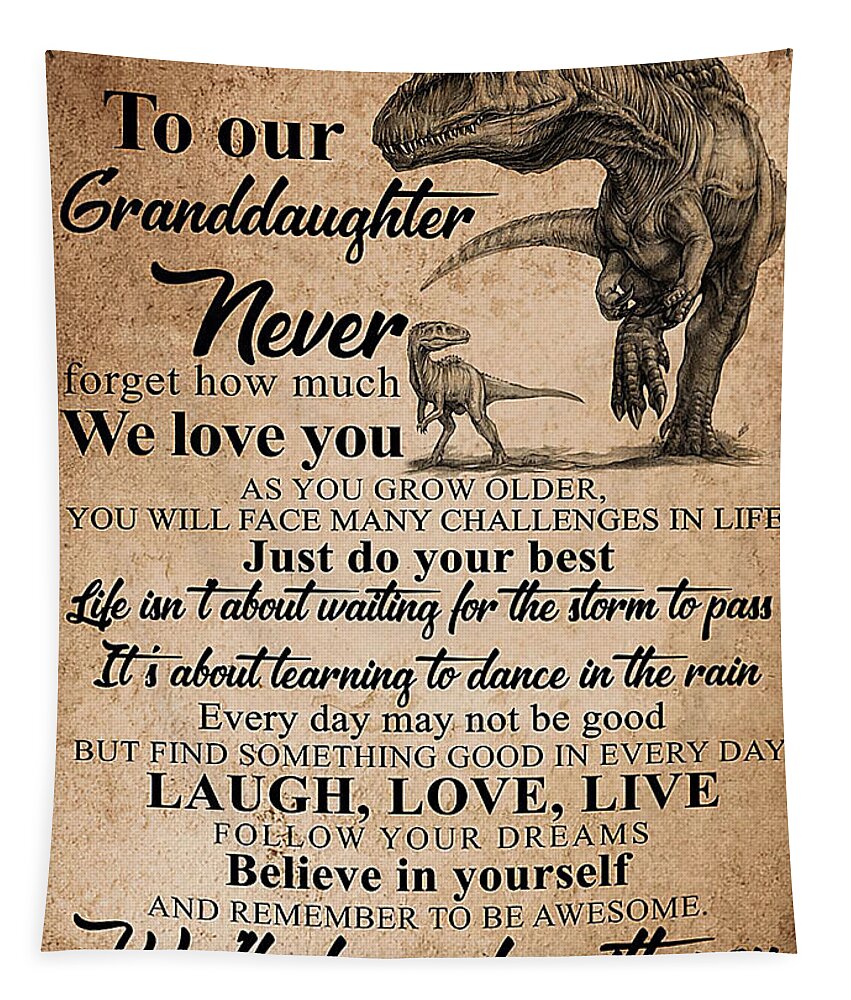The image depicts a heartfelt message to a granddaughter set against a light brown, tannish background. Dominating the upper right corner are illustrations of a small and a large T-Rex, rendered in black and white. The larger T-Rex, presumed to represent the grandparent, is partially cut off at the top, missing its eyes while looking off to its right. The smaller T-Rex gazes up at the larger one. The message, written in varying sizes and styles of Arial font—some in all capital letters and others not—begins in the upper left corner and flows down alongside the dinosaurs, eventually filling the page. It reads: "To our granddaughter, never forget how much we love you. As you grow older, you will face many challenges in life. Just do your best. Life isn't about waiting for the storm to pass. It's about learning to dance in the rain. Every day may not be good, but find something good in every day. Laugh, love, live, follow your dreams, believe in yourself, and remember to be awesome." At the very bottom of the image, there are fragments of additional letters, slightly cut off, hinting at more text beyond view. This picture has the appearance of a card or poster and might possibly be a product image like one you would find on an online shopping site.